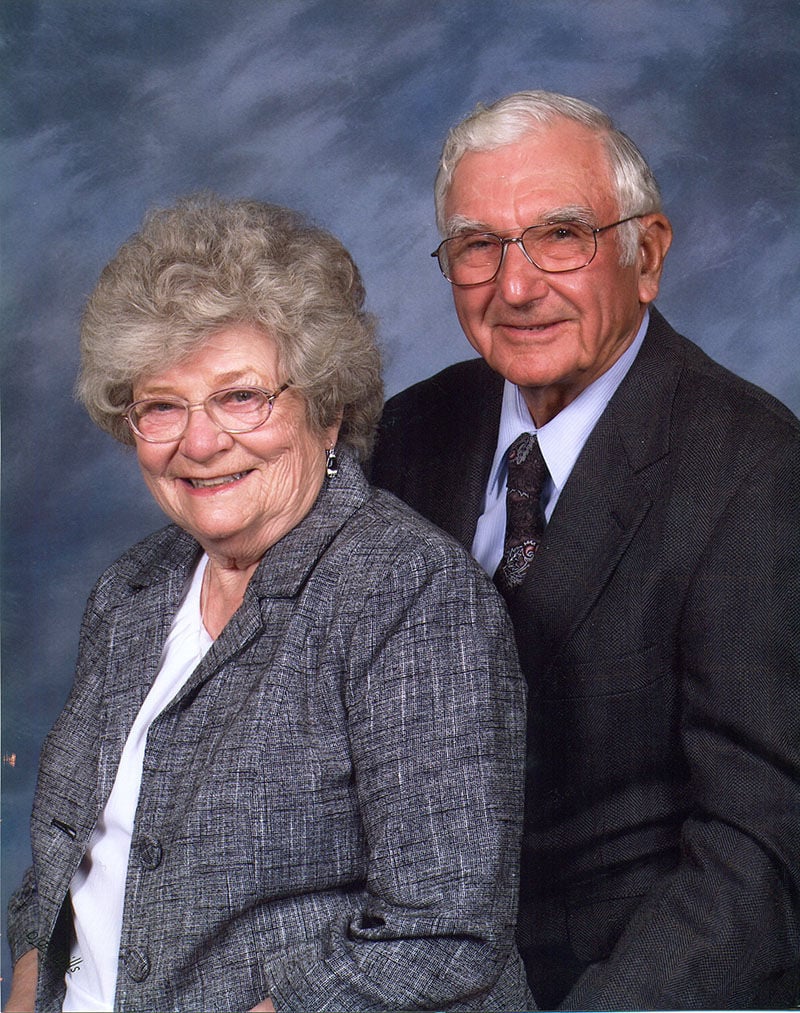This is a detailed portrait photograph of an elderly white couple set against a bluish-gray, smoky-patterned backdrop reminiscent of children's yearbook photos. The man, positioned slightly behind the woman, has short white hair and glasses, and he is dressed formally in a dark suit with a light blue undershirt and a black patterned tie. The woman, standing or seated just in front of him, is also wearing glasses, and her gray hair is styled in a poofy, curled manner. She is dressed in a gray tweed blazer with a white or light blue blouse underneath. Both individuals are smiling warmly at the camera, presenting a classic, affectionate pose.